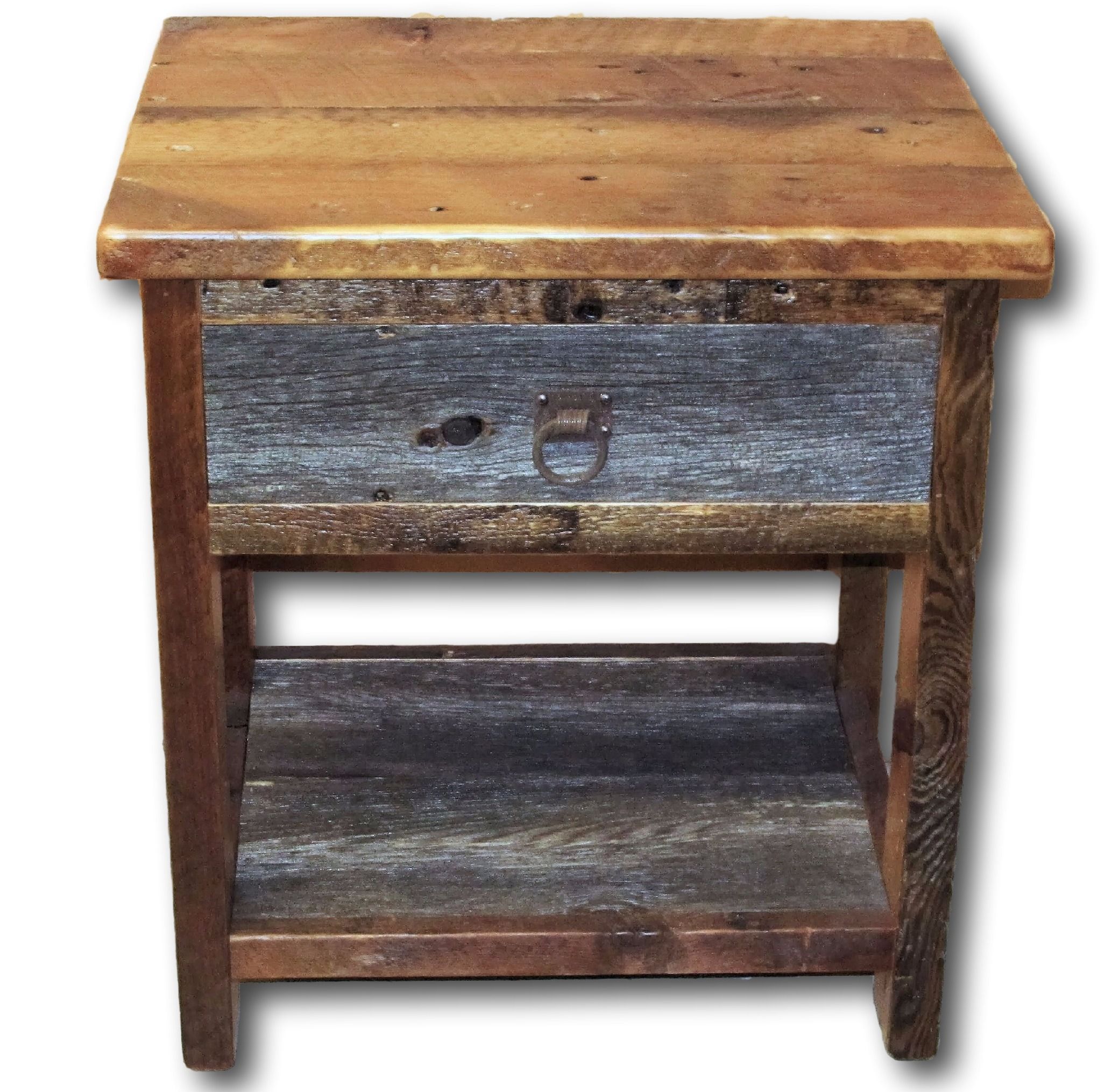This image showcases a rustic and slightly aged wooden night table. The table features a nicely sanded and finished pine top with slightly rounded edges and corners, presenting a light, worn appearance indicative of use over time. The legs of the table are a medium-toned pine, complementing the lighter top. The front of the table highlights a drawer made to look like reclaimed barn wood, with a grayish tone invoking a sense of history and texture. The drawer is adorned with a metal circular pull ring, adding to the vintage charm. Surrounding the drawer are plank woods of varying tones, including darker brown frames that are finely finished. Below the drawer is an open shelf framed by the same darker brown wood, providing additional storage or display space. Overall, the table's mixed wood tones and aged finishes give it a charmingly rustic appearance, set against a transparent or white background.